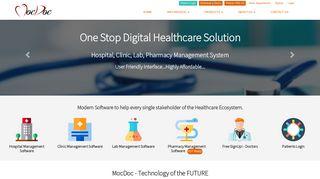The image is a small, detailed screenshot of the homepage for a digital healthcare management system. At the top of the page, prominently displayed in a banner, are the words "One Stop Digital Healthcare Solution," followed by an elaboration indicating that it serves as a "Hospital, Clinic, Lab, Pharmacy Management System." Although some of the text is too small to discern clearly, the main elements stand out. 

Beneath the banner, there are several icons representing different aspects of healthcare: a hospital, a laboratory, and a pharmacy. These icons have a cartoon-like, computer-generated design. The main banner features a stethoscope lying on a counter, which cleverly forms part of the site's name, "MocDoc."

Text at the bottom of the banner reads "MocDoc: Technology of the Future." The site’s overall color scheme includes a light gray or white background with some buttons highlighted in orange. Though there are additional links at the top of the homepage, the text is too small to read in this image.